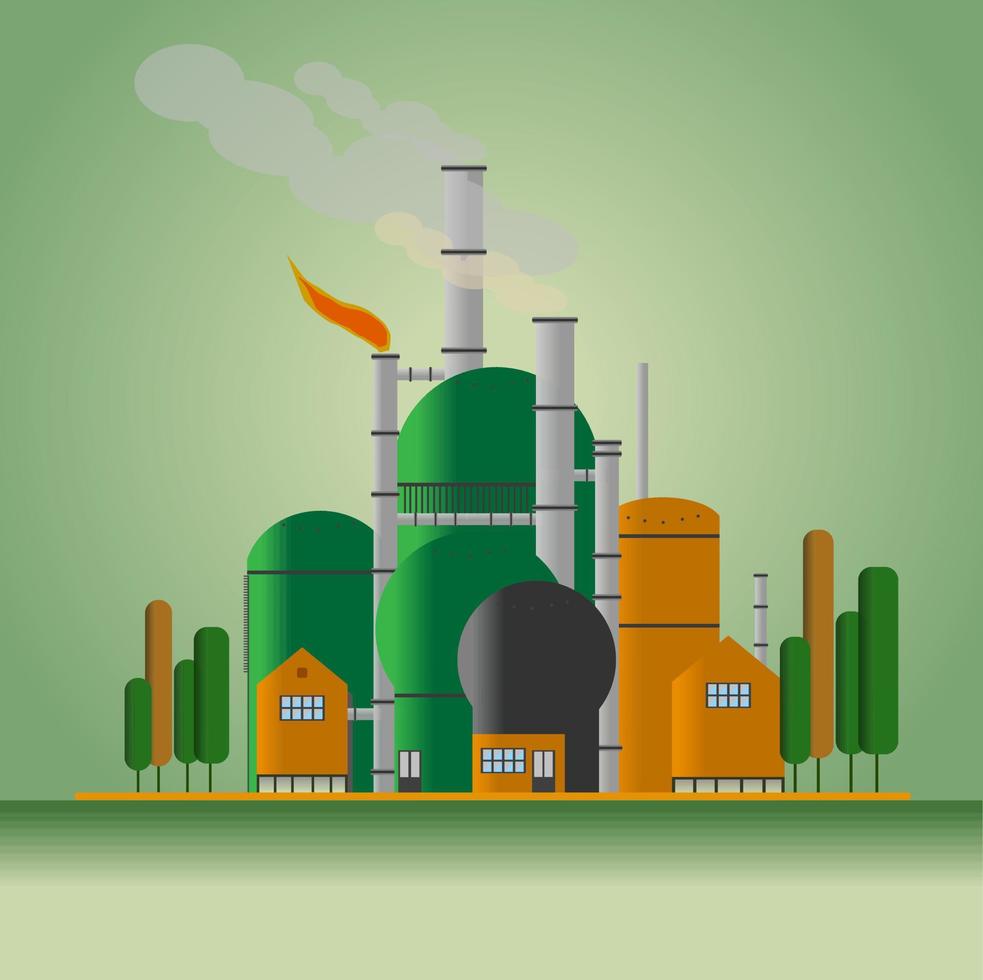The image appears to be a stylized digital artist's rendition of a chemical plant or industrial manufacturing facility. The scene features simplified structures with a color palette of friendly green, orange, and some black. Dominating the layout are large green cylindrical tanks topped with spherical domes, and interconnected gray smokestacks or distillation towers, some with smoke and flames emanating from their tops. There are also several orange rectangular buildings with windows, contributing to an industrial yet oddly inviting aesthetic. The plant is situated against a gradient light green background, flanked by minimalist, lollipop-like trees in green and orange, enhancing the scene's surreal and almost propagandistic portrayal of industrial activity in harmony with nature.